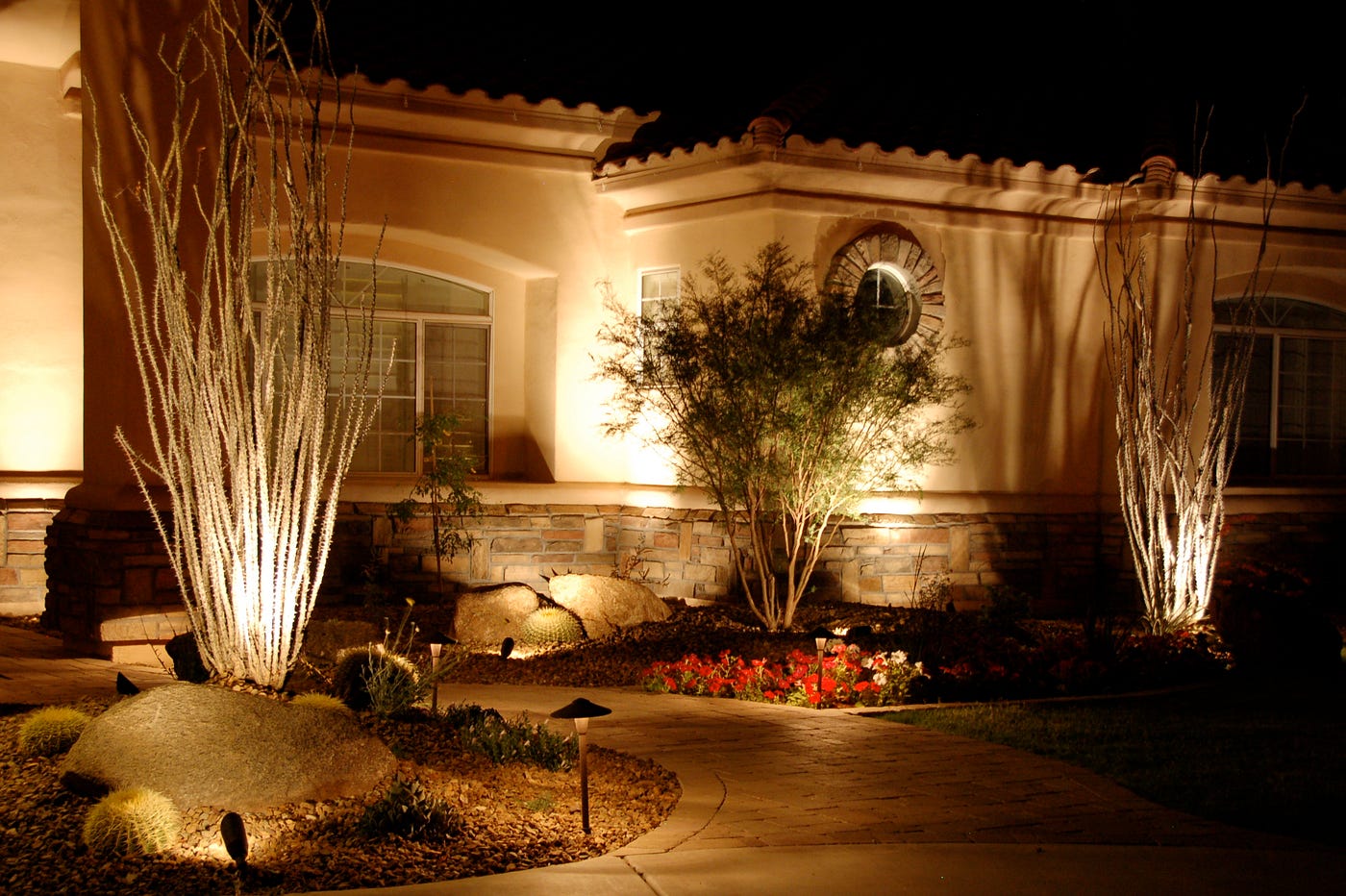This color photograph, taken at night, captures a single-story, potentially fancy building with a distinctive, well-lit exterior. The building features a curved brick walkway adorned with small nightlights and lamps embedded within the surrounding flower gardens. The garden's diverse flora includes a prominent large round cactus, peculiar dead-branch-type plants, and a vibrant mix of red, yellow, and white flowers positioned at the corner. Scattered large boulders further enhance the landscape. Although the building’s exact purpose is unclear—ranging from a house to possibly a nursing home or hospice—the image clearly showcases its elegant design and meticulously maintained outdoor space.